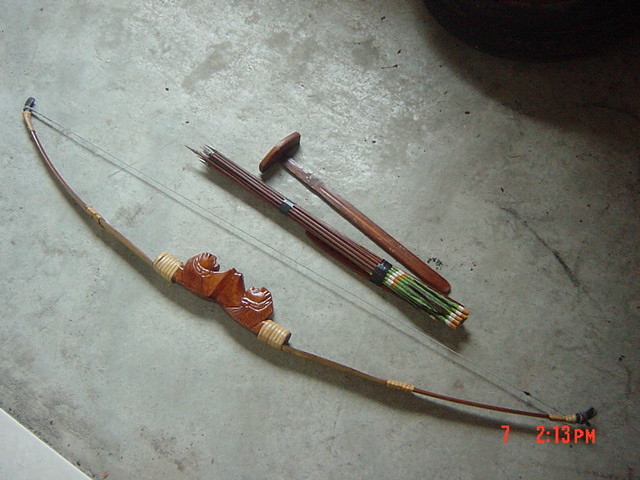This overhead color photograph captures a detailed scene featuring a bow and its accompanying quiver of arrows. The bow, made of wood and featuring a reddish center adornment, is shaped in a curved design. Its thin string, tightly wound, stretches across from one side to the other. Next to it lies a quiver containing arrows bound together, exhibiting a dark brown tip and a base colored in green, white, and orange. The arrows and quiver share a brownish tone. They are positioned diagonally on a drab, gray stone floor, pointing from the lower right to the upper left corner. Adjacent to this, there is a pedestal-like object of similar brown hue. A shadowy dark ball or object is visible in the top right corner. At the bottom right of the photograph, a red time stamp indicates 7 to 13 p.m.